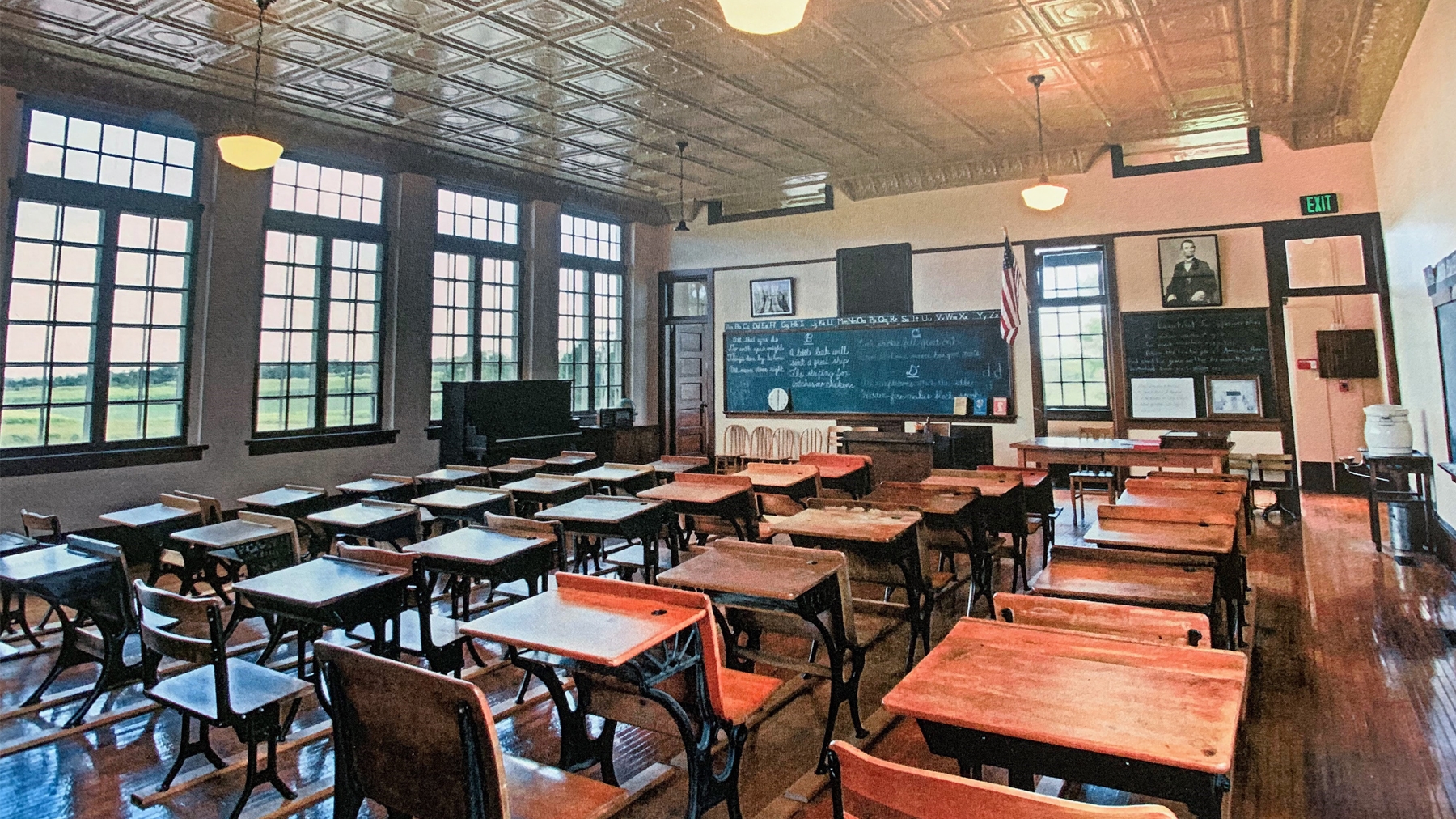The image depicts a vintage classroom with a wooden floor and ornate pressed tin ceiling. The room features a series of black-framed, clear-pane windows on the left side, offering a view of grass and trees outside. At the front of the classroom, there's an old-fashioned chalkboard with a lot of writing, though the text is unreadable. To the right of the chalkboard, hangs a portrait of Abraham Lincoln with an exit sign above. The wall behind is a cream color. Below the chalkboard are several historical pictures and a table. A doorway with a wood door stands slightly open next to the chalkboard. On the left side of the room, a piano sits against the windows. The classroom is filled with rows of antique wooden desks with cast iron frames, arranged neatly. An American flag is displayed near the front of the room. The room is well-lit with various lights hanging from the ceiling. The colors in the room vary from shades of brown to light brown, gray, white, off-white, black, green, and orange. The photograph was taken from the back of the room during the daytime, capturing the full layout of the space, although no people are present.